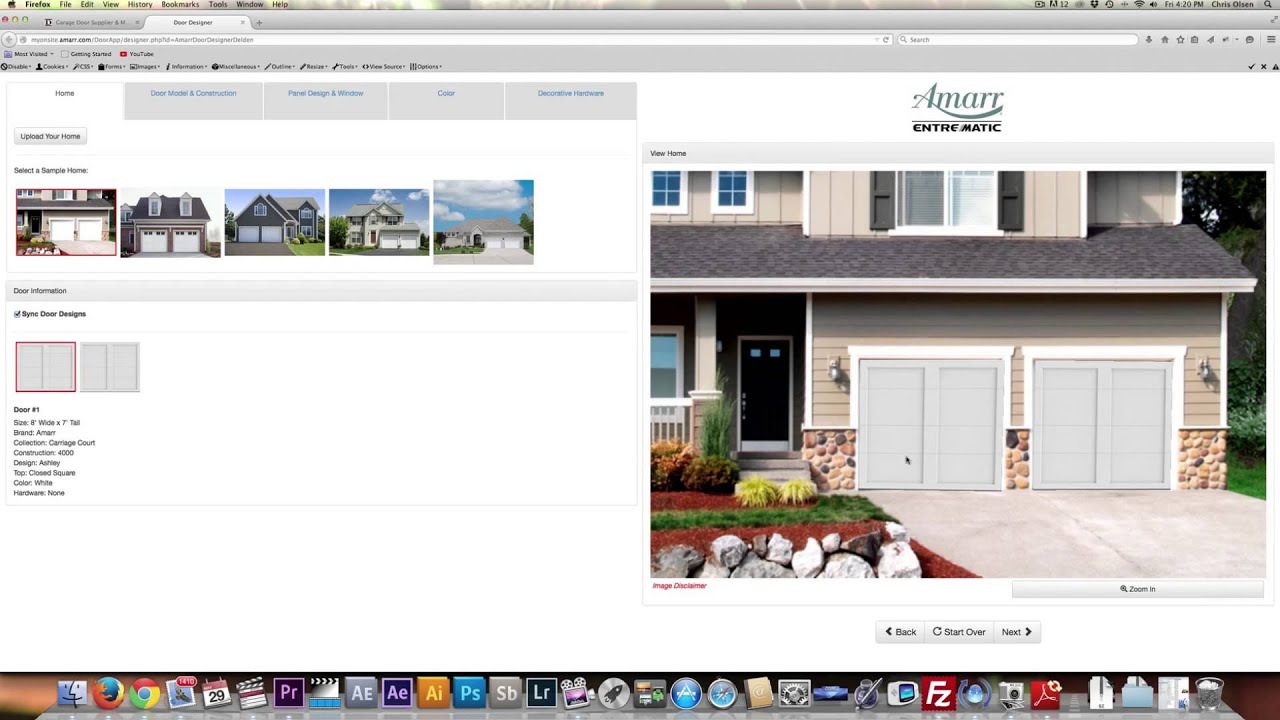The image features a user interface layout against a light purple backdrop at the top. The top section contains several tasks, some of which are crossed out, indicating completion. Below them, a long purple search bar sits above a white search box. Next, a row of titles spans across another purple line, followed by a white background area labeled "Home."

In this section, there are four small purple boxes, and labels that read "Amar" and "Traumatic" can be seen. A smaller purple button is positioned nearby. The main content area showcases five house images, each highlighting a beautiful house with a double garage. Underneath the images, there is a series of purple boxes, one of which is outlined in red, accompanied by text descriptions.

To the right, a large, captivating picture stands out: a stunning two-story house complete with a double garage, a well-manicured yard adorned with pretty rocks, a charming porch, and an inviting doorway. Above this picture, there's a light purple box. The bottom of this image features three buttons, accompanied by left and right arrow controls for navigation.

Finally, at the very bottom of the image, there's a vibrant, colorful box filled with various icons. These icons include a face, a globe, the Chrome logo, a magazine icon with a red tag, a calendar, and several others such as a purple AE, gray AE, yellow AI, blue PS, gray SH, gray LR, a camera, and a gray circle, among others. This bottom section is densely packed with diverse icons, adding visual interest to the interface layout.